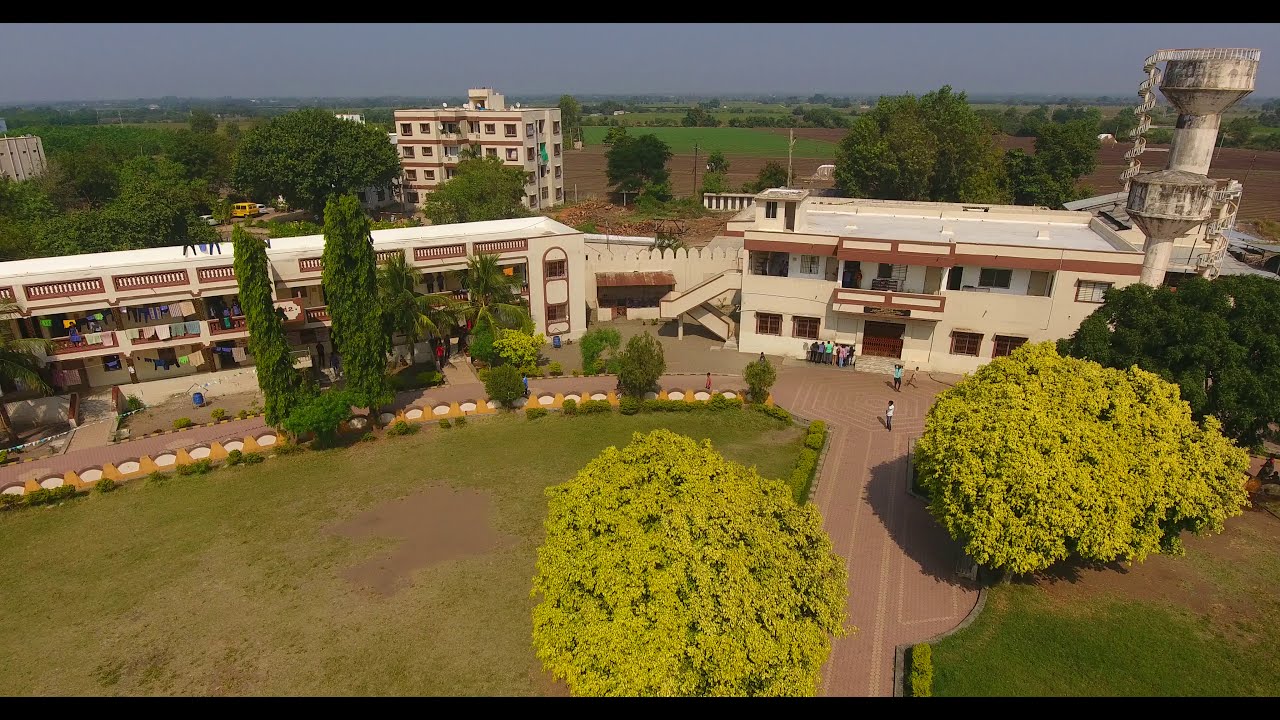This high-angle drone photograph captures a detailed view of what appears to be a small, well-maintained college campus or apartment complex. The central focus is on a wide, cream-colored building with dark brown borders. This two-floor structure is likely a dormitory, evidenced by the rows of balconies adorned with hanging laundry and people milling about. Surrounding the dormitory are neatly paved footpaths, vibrant green lawns, and clusters of bright green trees, contributing to a lively, springtime atmosphere.

In front of the building runs a brown pathway, with a gathering of people at the gates. A prominent feature near the building is an aged watchtower-like structure, possibly a water tank, adorned with black patches from years of weathering. The area also includes tropical palm trees, hinting at a warm climate, although the specific location is indeterminate.

To the right of the main building, an additional structure extends outward, further emphasizing the campus-style layout. The background reveals more apartment buildings of similar style, surrounded by expansive green spaces and fields, all under a clear, blue sky.